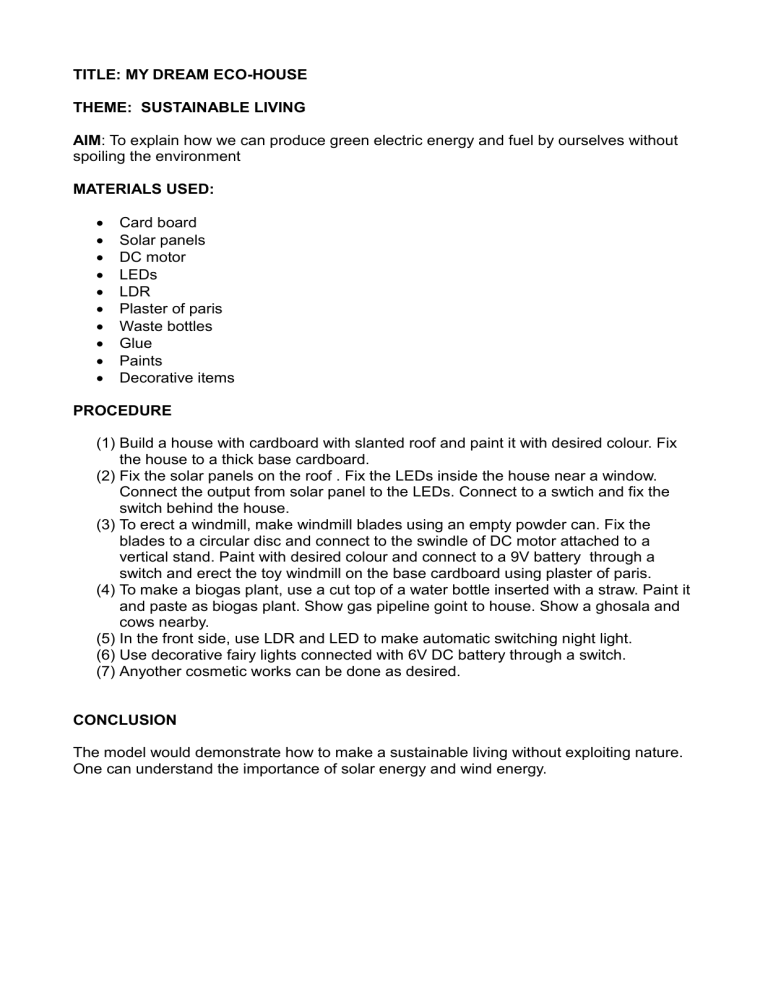### Caption:

This image captures a meticulously detailed sketch of someone's vision for building their dream house, styled uniquely like a resume. Titled "MY DREAM ECO HOUSE" in bold, all-capital letters at the top, the document lays out a clear framework for a project centered around sustainable living. 

The theme, stated as "Sustainable Living," is followed by the aim: "To explain how we can produce green electric energy fuel by ourselves without spoiling the environment." The sketch lists the materials required for this eco-friendly house, including cardboard, solar panels, a DC motor, LEDs, an LDR (Light Dependent Resistor), plaster of Paris, waste bottles, glue, paints, and various decorative items.

Beneath the material list, the document methodically explains the building procedure in five steps. Step one involves constructing a house with a slanted roof out of cardboard and painting it in the desired color. The house is then affixed to a thick base made of cardboard. As the steps progress, it details how to erect a windmill by crafting blades from an empty powder can and attaching them to a circular disc connected to the spindle of a DC motor.

The detailed sketch serves as a comprehensive guide, illustrating a model for a sustainable living environment using renewable energy sources, such as windmills, effectively integrating green practices into home building.